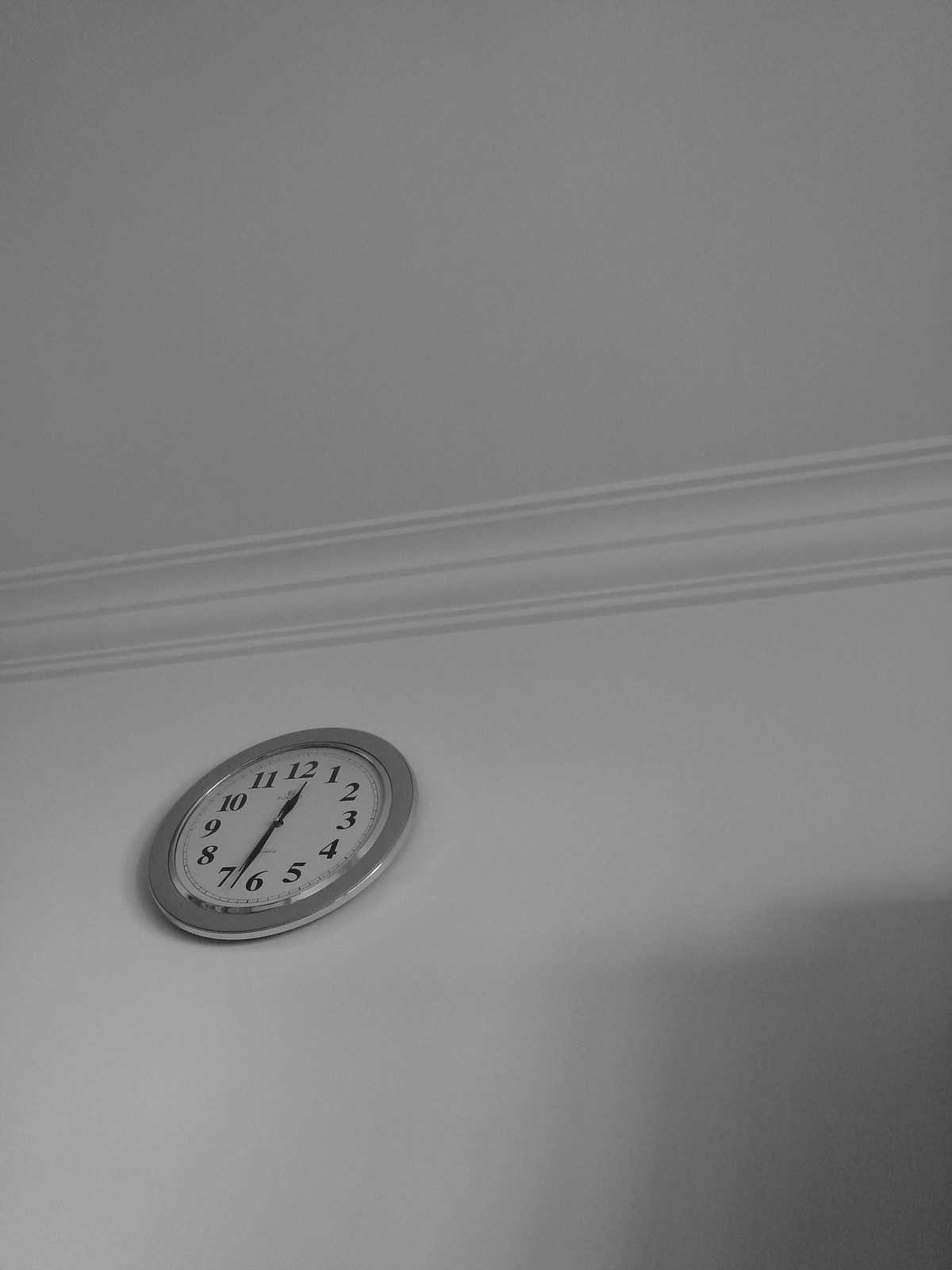This photograph captures the interior of a room, showcasing a prominently featured wall clock positioned against a stark white wall. The clock itself has a large, thick silver bezel and a pure white face marked with black numbers in the standard 1-through-12 typeset. Black hands — specifically an hour and a minute hand, but notably without a second hand — point to a time around 12:32 or 12:33. Tiny black lines serve as minute markers between the numbers. The photo, taken from below at an angle, distorts the clock slightly to look oval-shaped. The lower right-hand corner of the image contains a blurry, dark gray section, possibly a soft-edged shadow. Above the clock, white crown molding with distinct ridges and curves transitions into the ceiling, emphasizing the room's clean, orderly appearance. This clean and detailed black-and-white image captures a simple yet elegant piece of timekeeping against minimalistic decor.